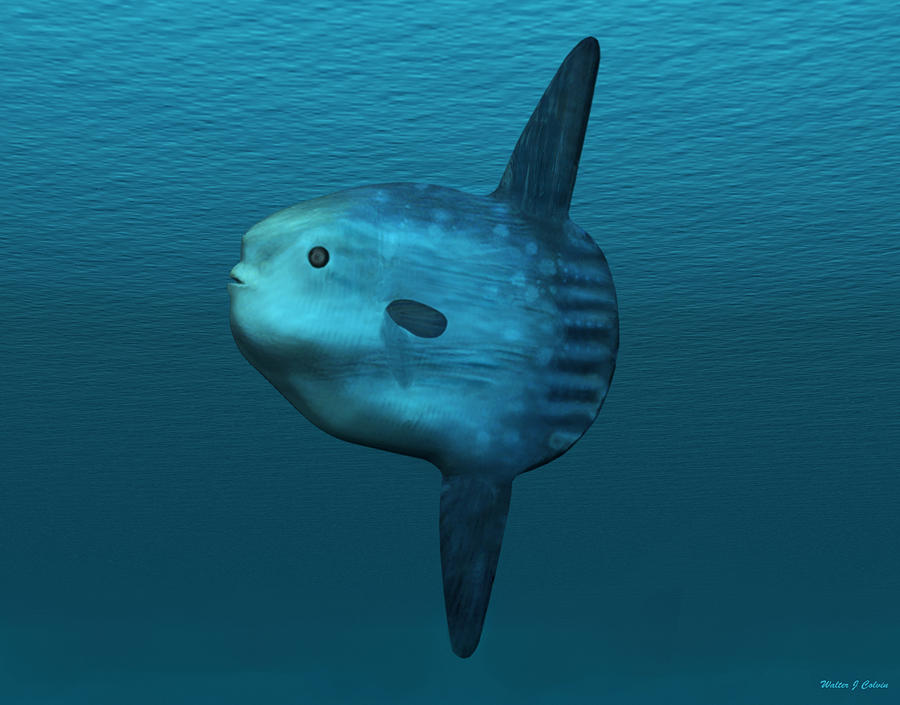The image features a peculiar, broad, and flat fish situated underwater, with a textured water surface visible above. The water background transitions from a lighter blue at the top to a darker, murkier blue towards the bottom. The only object in the image, the fish faces left and appears quite flat, akin to the palm of a hand. It has a slightly humanoid face with a sloped nose and a small, protruding mouth. Its round, large eye is clearly depicted, conveying an almost lifelike quality.

The fish's body exhibits a gradation of colors, starting with an aqua hue at the head, moving to a darker blue in the middle, and culminating in a navy shade towards the tail. Light blue and white speckles create a patterned appearance against its grayish-blue body. The fins are darker blue compared to the body, with a prominent shark-like dorsal fin and a matching ventral fin underneath. Both fins are positioned symmetrically towards the rear. The tail is distinctively flat and paddle-like, not tapering but maintaining the same width as the rest of the fish.

Additionally, the fish has light patches and dark stripes interspersed with spots, enhancing its textured look. At the bottom right corner of the image, there's an illegible, minuscule watermark signature.